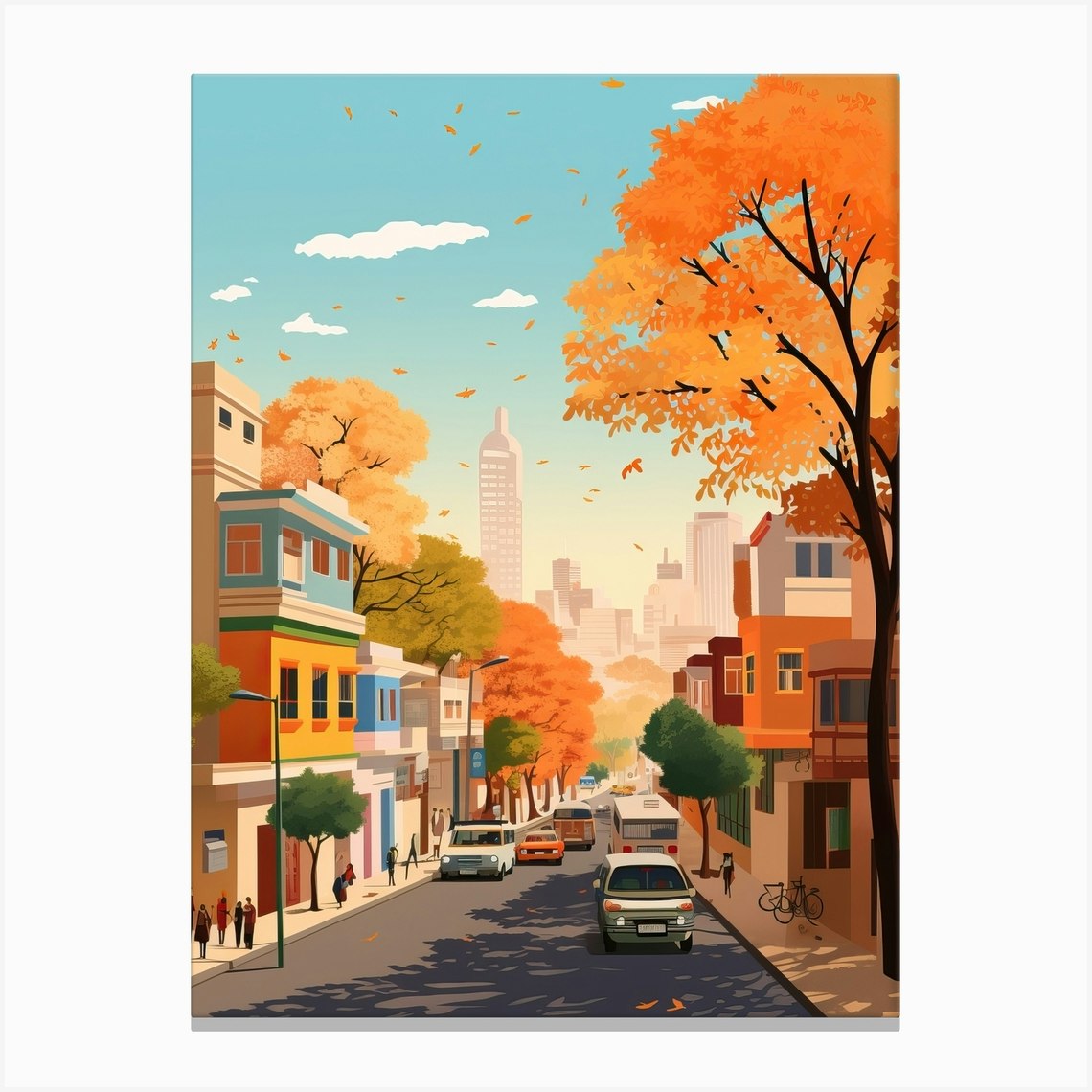The illustration portrays a vibrant city street in autumn, descending towards a distant skyline of tall, gray skyscrapers. The sky above is a bright blue with a few thin, wispy clouds. The roadside is framed with trees in various stages of fall, exhibiting a spectrum from green to yellow and vibrant orange, with leaves drifting down from branches. The trees have distinct thin black trunks, and the orange leaves appear especially prominent on the right side of the road.

The foreground is bustling with activity: colorful buildings with block designs line the street, displaying hues of blue, green, and yellow. Notably, the top story of a building on the left is blue, followed by a yellow story with a green roof and orange window frames. Pedestrians populate the sidewalks, more densely on the left side, and there's a bike parked alongside one of the buildings. Various vehicles, including cars, buses, and a possible minivan, travel the street, while lampposts and streetlights add detail to the urban scene. Shadows from the trees cast upon the pavement, enhancing the dynamic fall atmosphere. Overall, it's a clean, colorful, and active cityscape painting, signed by an artist, adding a personal touch to the lively urban depiction.